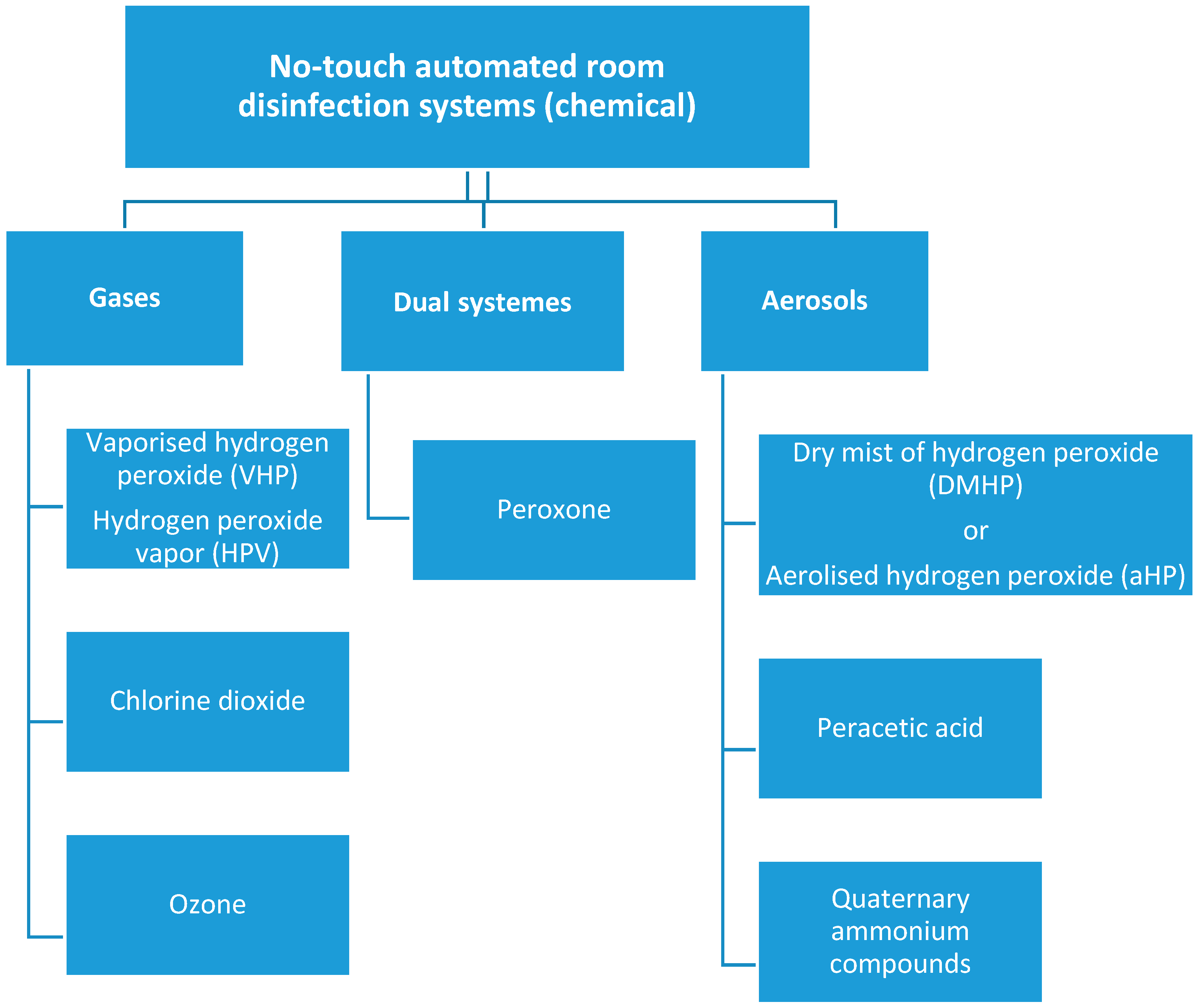The image displays a detailed flowchart of a no-touch automated room disinfection system using chemical agents. The design features a bright blue color scheme with white font. At the top, the main box is labeled "No-Touch Automated Room Disinfection Systems (Chemical)." 

Below the main box, two short vertical lines lead to a horizontal line that branches into three sections, each with its own dark blue rectangle. The left rectangle is labeled "Gases," the center is labeled "Dual Systems," and the right is labeled "Aerosols."

From the "Gases" box:
- It branches downward into three vertically stacked blue rectangles.
  - The first rectangle is labeled "Vaporized Hydrogen Peroxide (VHP)" and "Hydrogen Peroxide Vapor (HPV)."
  - The second rectangle below it says "Chlorine Dioxide."
  - The third and final rectangle says "Ozone."

From the "Dual Systems" box:
- A single line goes downward to one rectangle labeled "Peroxone."

From the "Aerosols" box:
- It connects downward to two vertically stacked blue rectangles.
  - The first rectangle is split into text labels: "Dry Mist of Hydrogen Peroxide (DMHP)" and "Aerolyzed Hydrogen Peroxide (AHP)."
  - The second rectangle below it says "Parasitic Acid."
  - The final rectangle in this column states "Quaternary Ammonium Compounds."

Thin blue lines connect all the boxes and maintain a structured and hierarchical layout, ensuring clarity in the flowchart's structure and process depiction. The chart utilizes British English spelling, notably replacing "Z" with "S" in words like "systems."